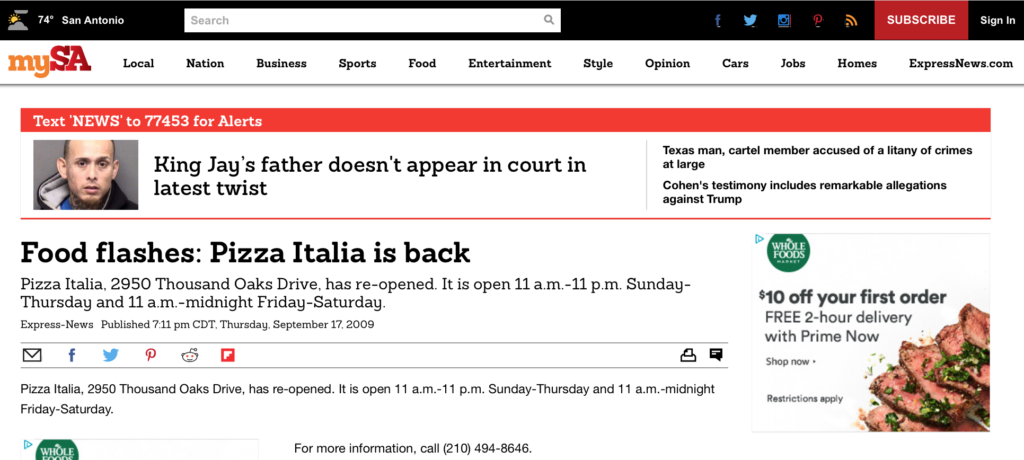The image depicts a webpage with a black border at the top. Displayed prominently at the top of the border is the text "74 degrees, San Antonio." Below this temperature information, the site features a navigation bar listing various sections: "My SA," "Local," "Nation," "Business," "Sports," "Food," "Entertainment," "Style," "Opinion," "Cars," "Jobs," "Homes," and "ExpressNews.com."

A vibrant red box stands out on the screen, urging users to "Text NEWS to 774534 for alerts." 

The main headlines displayed on the page include:
1. "King Jay's father doesn't appear in court in latest twist."
2. "Texas man, cartel member accused of a litany of crimes, at large."
3. "Cohen testimony includes remarkable allegations against Trump."
4. "Food Flashes: Pizza Italia is back! Pizza Italia at 2950 Thousand Oaks Drive has reopened. It is open 11 a.m. to 11 p.m. Sunday through Thursday and 11 a.m. to midnight Friday through Saturday. Express News published this article at 7:11 CDT on Thursday, September 17, 2009."